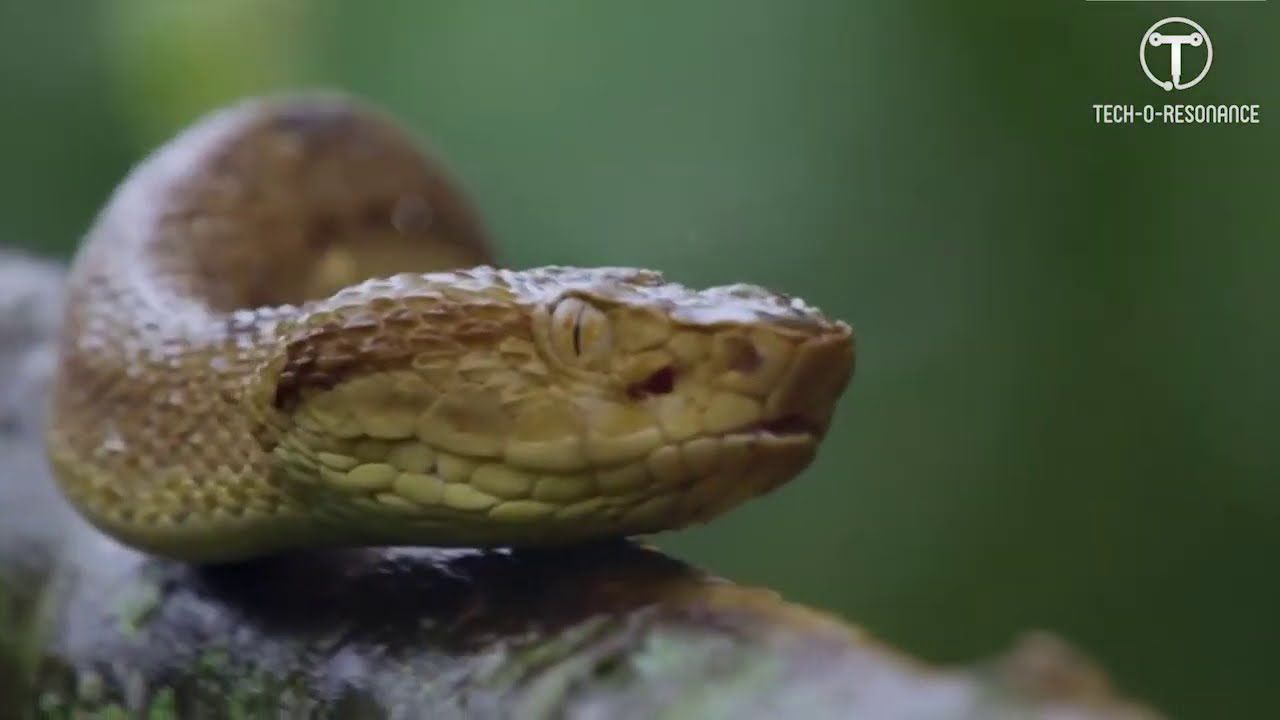In this close-up image, a snake is positioned prominently atop a tree branch, which appears dark in color and is textured with small green patches, possibly from foliage or moss. The snake's head is situated towards the left and points to the right, displaying a vertically slit eye. The visible portion of its sinuous body extends to the right, forming an 'S' shape before disappearing from view. The snake's scaly skin is a blend of brown, golden, and gray hues, with certain parts appearing almost off-white. Its mouth is closed, giving it a serene expression. The background is a blurred mosaic of green, suggesting a lush forest or jungle setting. In the upper right corner of the image, there is a T inside a circle, accompanied by the text "Tech-O Resonance."